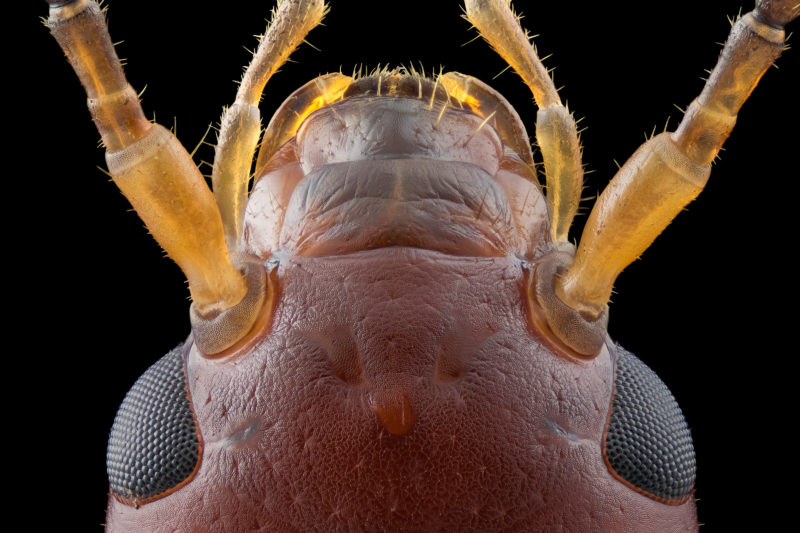The image is an up-close capture of an insect, likely an ant, prominently showcasing its intricate head. The insect head is a reddish-brown color, tapering towards the mouth. Its compound black eyes, each resembling a cluster of tiny boba balls, are bordered by an orange ring. Delicate, light brownish-orange antennas, with a translucent quality and sparse hair, emerge from either side of the head and mouth area. The head also features a black section at the top, adding contrast. The insect’s 'shoulders' have a textured appearance, akin to that of a basketball, characterized by numerous dimples. Adding a touch of moisture, a water droplet is perched on its forehead, and the insect is set against a stark black background.